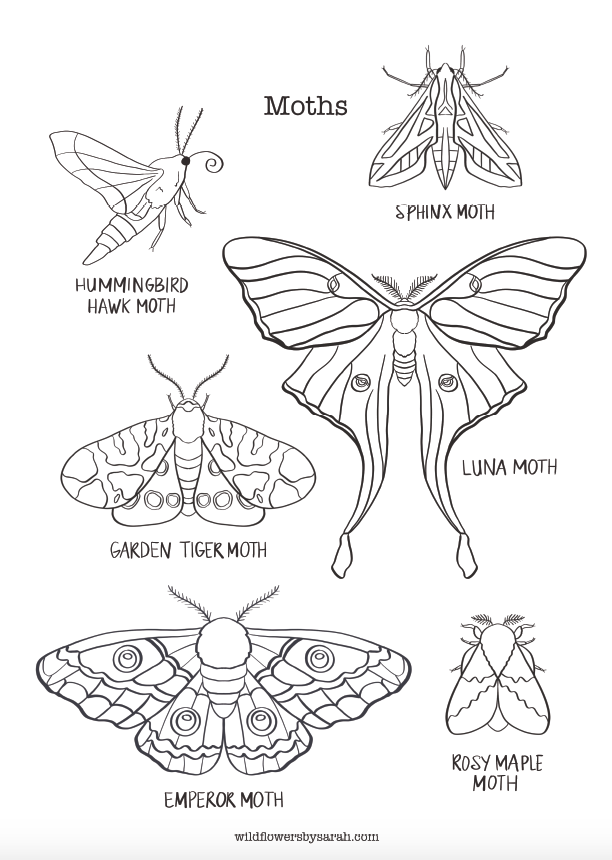The vertically oriented, black and white image showcases detailed hand-drawn illustrations of six different kinds of moths on a white background, emphasizing their distinct shapes and wing patterns. Centered at the top, the word "MOTHS" is prominently displayed in black letters. To the left of this title is a hummingbird hawk moth, and to the right, a sphinx moth. The largest moth, the luna moth, noted for its long, tail-like extensions on its wings and fern-like antennae, is positioned prominently. Adjacent to the luna moth is the garden tiger moth. The bottom row features an emperor moth on the left, identifiable by the unique circles on its wings, and the smallest among them, the rosy maple moth, on the right. The illustrations are strictly monochromatic, focusing on form and design rather than color. At the bottom of the poster is the website "whiteflowerbysara.com."